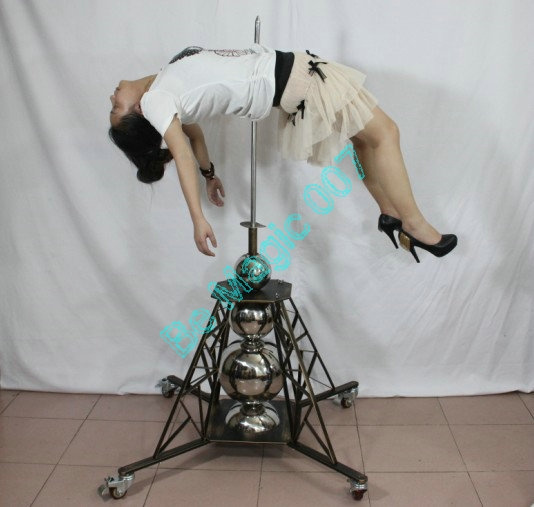The photograph showcases a dramatic scene involving a woman staged against a white cloth backdrop, suggesting a magic act given the text overlay "Be Magic 007" in teal and cyan font. The woman, who appears to be of Asian descent, has dark hair and is dressed in a white t-shirt, a brown ruffled skirt with black bows, and black high heels. She is impaled through the abdomen by a vertical, spear-like spire protruding from a tower-like black stand with silver accents. Her back is arched, her chest faces upwards, and her legs point towards the ground, creating a visually striking and intense image. The scene is set on a beige taupe tiled floor, further enhancing the starkness of the dramatic tableau.